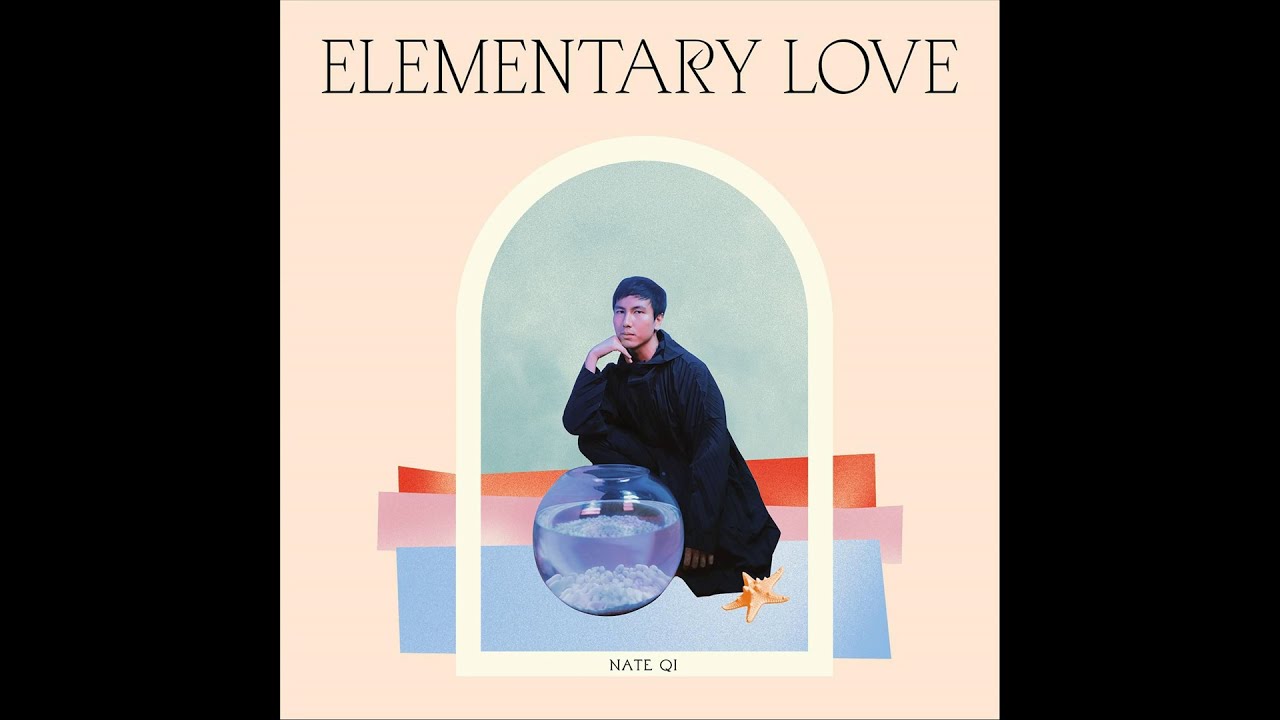The image appears to be an album cover set within a horizontal rectangular frame, flanked by thick black borders on the left and right sides. The central, square portion features an off-white arch against a pale pink background. At the top of the image, in large black capital letters, the text reads "ELEMENTARY LOVE." Inside the archway, there's a mixed-color backdrop consisting of a pink rectangle at the top, a crooked red rectangle beneath it, and a thick blue band at the bottom.

The focal point within the arch is an illustration or photograph of an Asian man with short black hair, dressed in a long black robe resembling a monk's or a judge's cloak. He is in a contemplative pose, squatting with his right elbow resting on his knee and his chin propped on his right hand. In front of him sits a fishbowl containing some white elements but no fish. An orange starfish is located at the bottom right near the end of his robe.

Additionally, there is some black text, possibly reading "Nate Key," at the base of the white archway, although it is not entirely clear. The overall composition and color scheme with its striking contrasts convey a blend of simplicity and thoughtfulness.